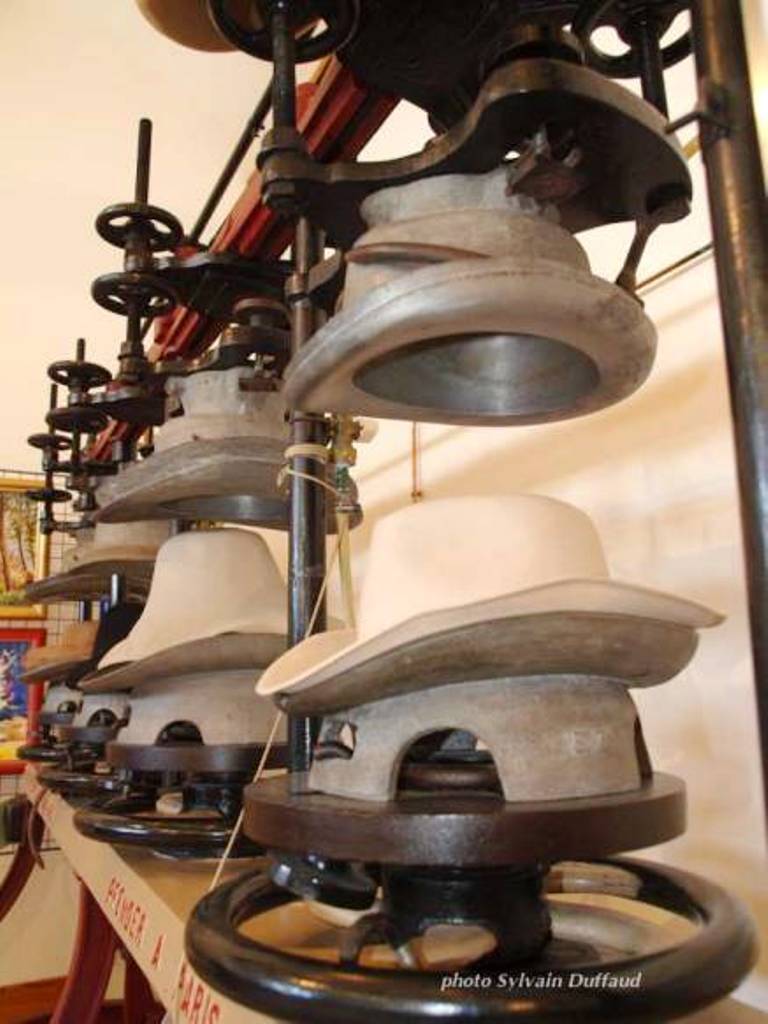The image portrays an industrial hat-making workshop, likely in France or a French-speaking country, as indicated by the text "à Paris" on the machinery and "photo Sylvain Duffod" in the bottom right corner. Central to the image are several metal forms and stands used for shaping hats. The process appears to be depicted in various stages, with two white hats visibly in production. One of these hats looks nearly completed, while the other is still being shaped. The machinery functions by pressing the material up into molds to form the hats, resembling an assembly line. The workspace features a table with red legs, white walls, and a mix of metal and red machinery components, emphasizing the industrial nature of the hat-making process.